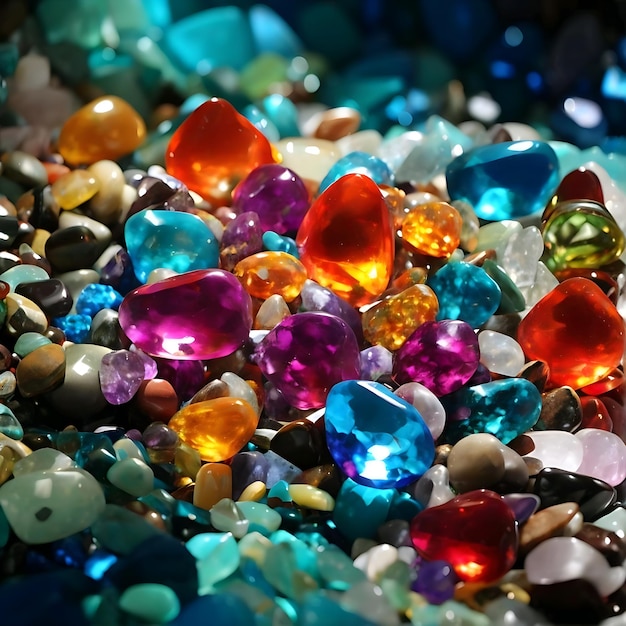The image showcases a vibrant collection of glossy and shiny rocks, resembling gems or crystals, filling the entire frame. The rocks vary in size from very small to medium and come in a dazzling array of colors, including clear white, pink, turquoise blue, darker blue, purple, several hues of orange and red, black, and white. The rocks are piled on top of each other, their light-reflective surfaces adding to their jewel-like appearance. Larger rocks, particularly in purple, blue, and orange, are centrally placed, while some bright gold rocks can be seen on the far right. The background features a continuation of these colorful, variously shaped and sized stones, slightly blurred to emphasize the main set in focus. The high-quality image highlights the intricate details and diverse shapes, akin to marbles, enhancing the impression of a treasure trove of polished gemstones.